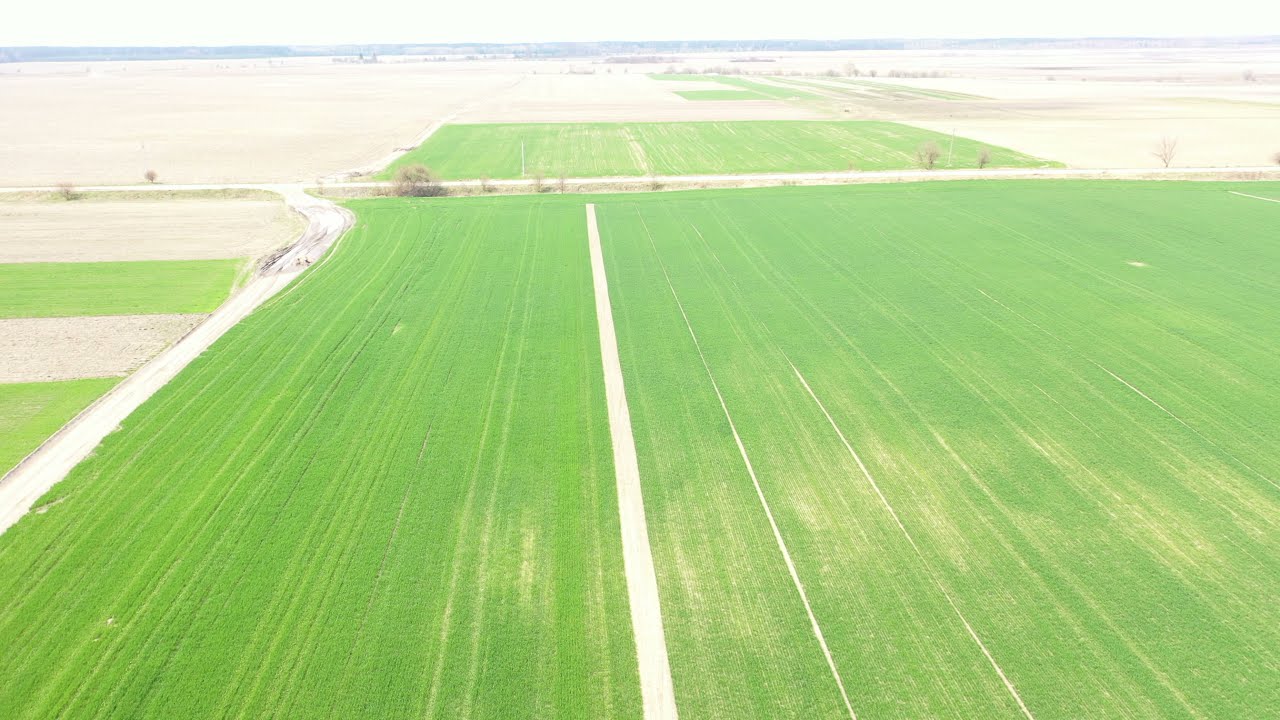The aerial image depicts an expansive, heavily lit landscape of farmland divided into large, rectangular fields of light and dark green. A distinct white road bisects the terrain vertically, while another road runs horizontally, segmenting the rear fields from the forefront. Alternating green and tan fields occupy the left side of the frame, contrasting sharply with the surrounding greenery. The fields are delineated by conspicuous, thick white lines. In the distance, light tan fields stretch towards the horizon, where a cloudless, gray sky meets the earth. A hint of water, possibly a river, ocean, or lake, shimmers in the background, further emphasizing the vast, open nature of the rural scene.